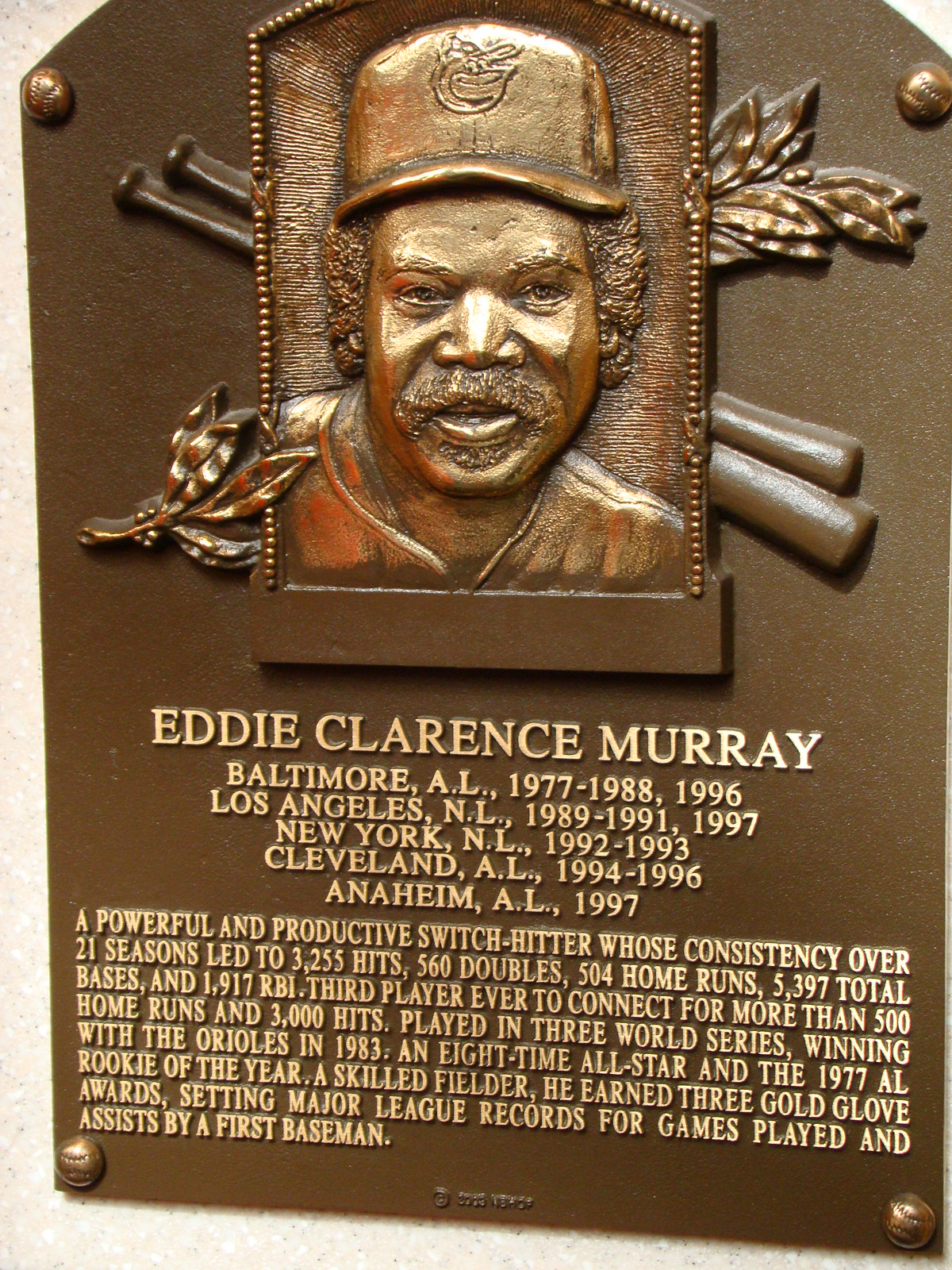The image depicts a detailed bronze plaque honoring Eddie Clarence Murray. Prominently featured in the center is an etched headshot of Murray, a distinguished African American baseball player, wearing a cap and displaying his characteristic mustache along with a small goatee, framed by bushy hair. Behind his head, two crossed baseball bats and gold-etched leaves adorn the plaque diagonally on either side.

Below the headshot, the text reads:
"Eddie Clarence Murray 
Baltimore AL 1977-1988, 1996 
Los Angeles NL 1989-1991, 1997 
New York NL 1992-1993 
Cleveland AL 1994-1996 
Anaheim AL 1997"

Further detailing his career highlights, the plaque states:
"A powerful and productive switch hitter whose consistency over 21 seasons led to 3,255 hits, 560 doubles, 504 home runs, 5,397 total bases, and 1,917 RBI. Third player ever to connect for more than 500 home runs and 3,000 hits. Played in three World Series, winning with the Orioles in 1983. An eight-time All-Star, and the 1977 AL Rookie of the Year. A skilled fielder, he earned three Gold Glove awards, setting major league records for games played and assists by a first baseman."

The bronze craftsmanship and detailed accolades encapsulate the remarkable career and legacy of Eddie Clarence Murray in Major League Baseball.